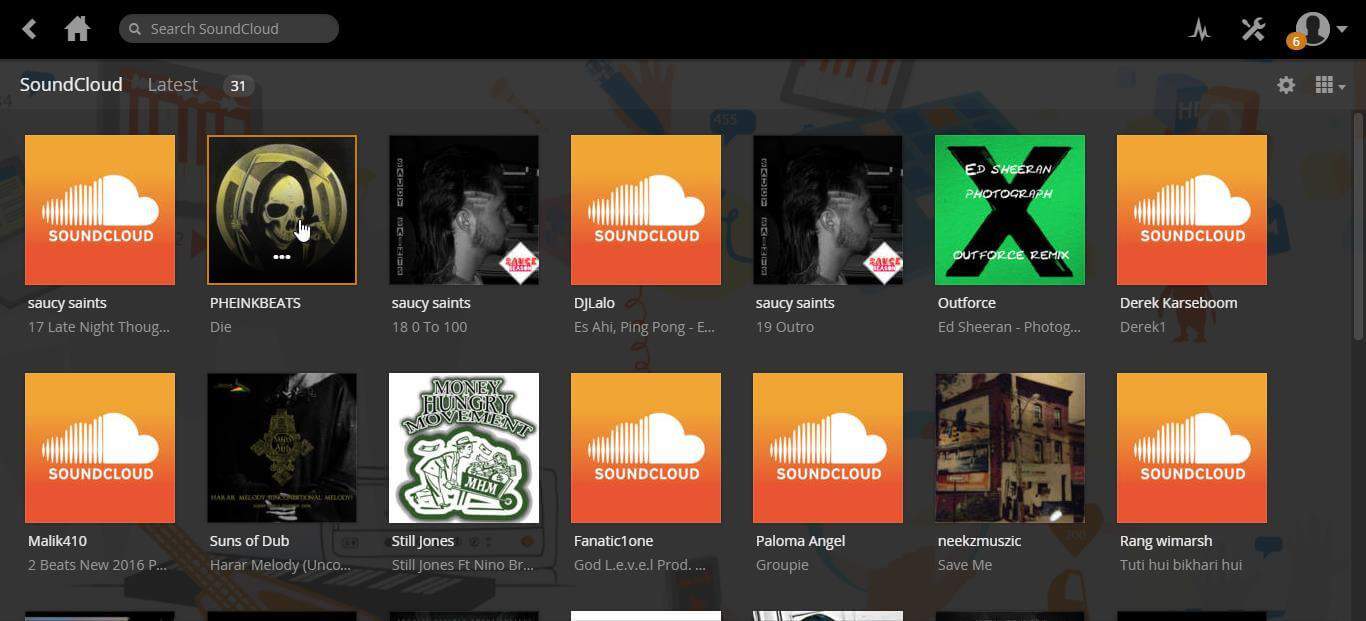A screenshot of a SoundCloud page is displayed, featuring a gray background with a prominent black bar at the top. Starting from the upper left, there is a left-pointing caret symbol next to a home icon. Adjacent to this is a search bar labeled "Search SoundCloud," accompanied by a magnifying glass icon. Moving to the upper right corner, there is a small logo resembling a segment of a bar or line graph. Next to it, crossed tools—specifically a wrench and a screwdriver—are visible. Further right, there is a user icon shaped like a silhouette of a person, with the number "6" in an orange circle superimposed on it.

Below the black bar, in the main body of the webpage, "SoundCloud" is written alongside the word "Latest" and the number "31." On the right side of this section, there is a settings gear icon followed by a 3x3 grid menu icon.

The page features two rows of album cover images, with a total of 14 square icons. Some album covers display unique artwork and artist names, while others are placeholders with the SoundCloud logo on a yellow and orange background. The top row showcases albums from artists such as Saucy Saints, Finkbeats, TJ Lalo, Outforce, Derek Kars, and Boom. The bottom row includes works from Malik 410, Sons of Dub, Still Jones, Phonetic One, Paloma Angel, Nyx Music, and Rang Why Marsh.